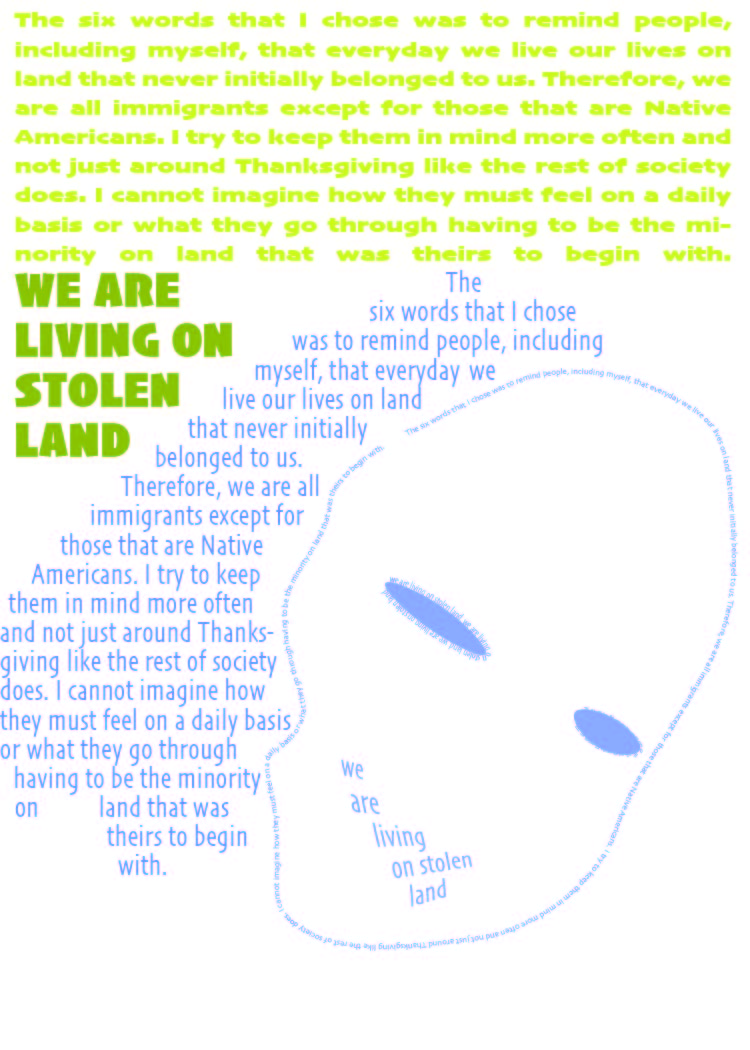The image features a powerful textual message spread across various sections. At the top, a medium-sized, yellow-green paragraph reads: "The six words that I chose was to remind people, including myself, that every day we live our lives on land that never initially belonged to us." Directly beneath this, in large, dark green capital letters, is a bold statement: "WE ARE LIVING ON STOLEN LAND." To the right, a paragraph printed in blue elaborates on the initial thought, saying: "The six words that I chose was to remind people, including myself, that every day we live our lives on land that never initially belonged to us." The right side of the image also features the outline of a human face, drawn in blue, with two blue eyes. Embedded within the mouth area, the phrase "WE ARE LIVING ON STOLEN LAND" is repeated in blue letters, emphasizing the core message. 

The whole composition consists exclusively of text and shapes that reinforce the critical reminder and reflection on the historical and ongoing realities of living on land that was originally inhabited by others.